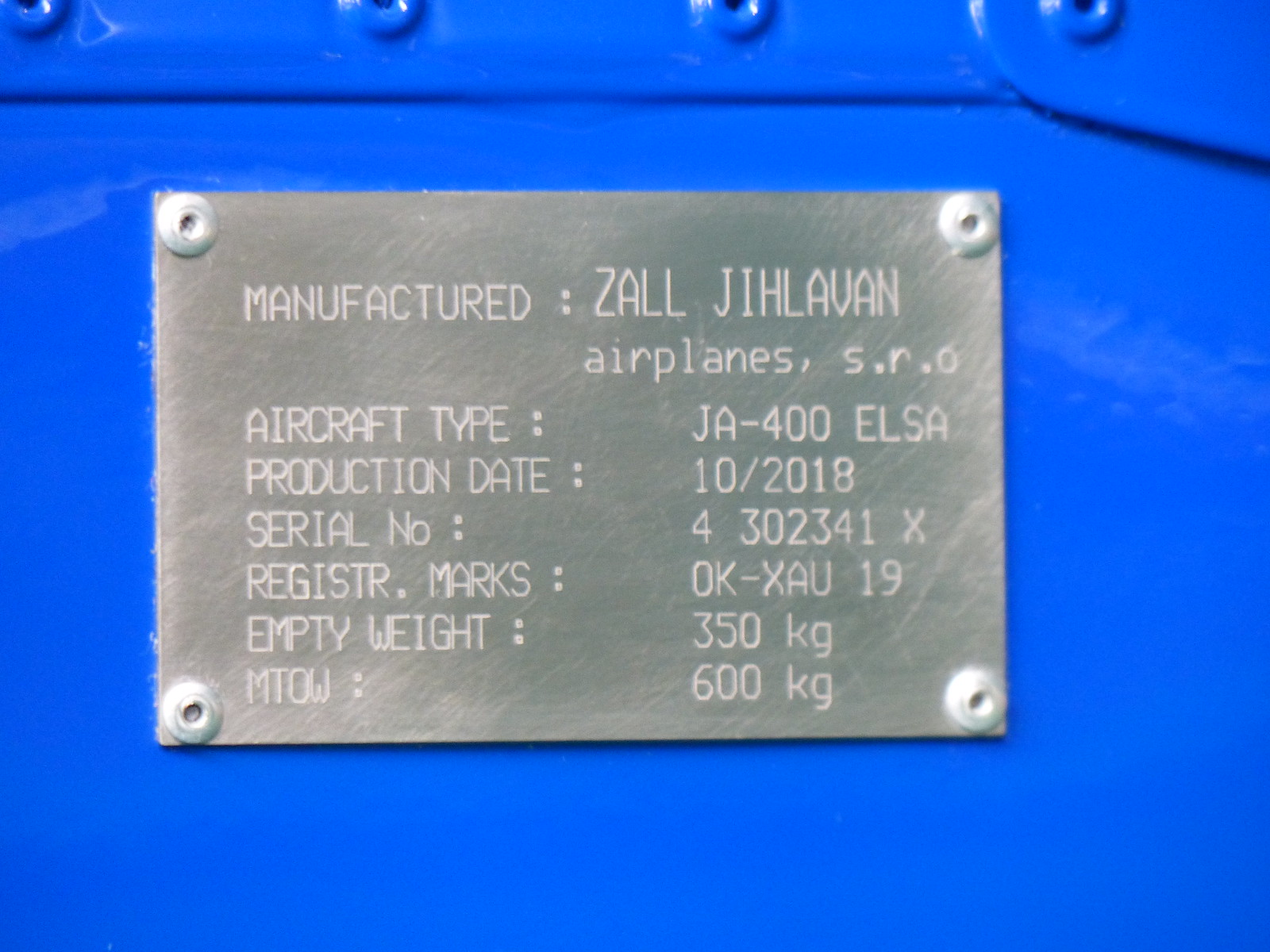The image features a close-up view of a vibrant, royal blue surface with bolts along the edges, some of which are slightly cut out of the frame. Mounted on this blue background is a grey metal placard with lighter grey bolts at each corner. The placard is stamped with detailed information. It reads, "Manufactured; CALL J-I-H-L-A-V-A-N. Below that, it states, "Airplanes, S.R.O." Further down, there are specific details listed in two columns. The left column contains labels: "Aircraft type," "Production date," "Serial number," "Registry Marks," "Empty weight," and "MTOW." Corresponding to these labels, the right column reads: "JA-400 ELSA," "10-2018," "4302341X," "OK-XAU-19," "350 kilograms," and "600 kilograms." The blue background is strikingly bright, reminiscent of an automotive finish, creating a sharp contrast against the metallic grey placard.